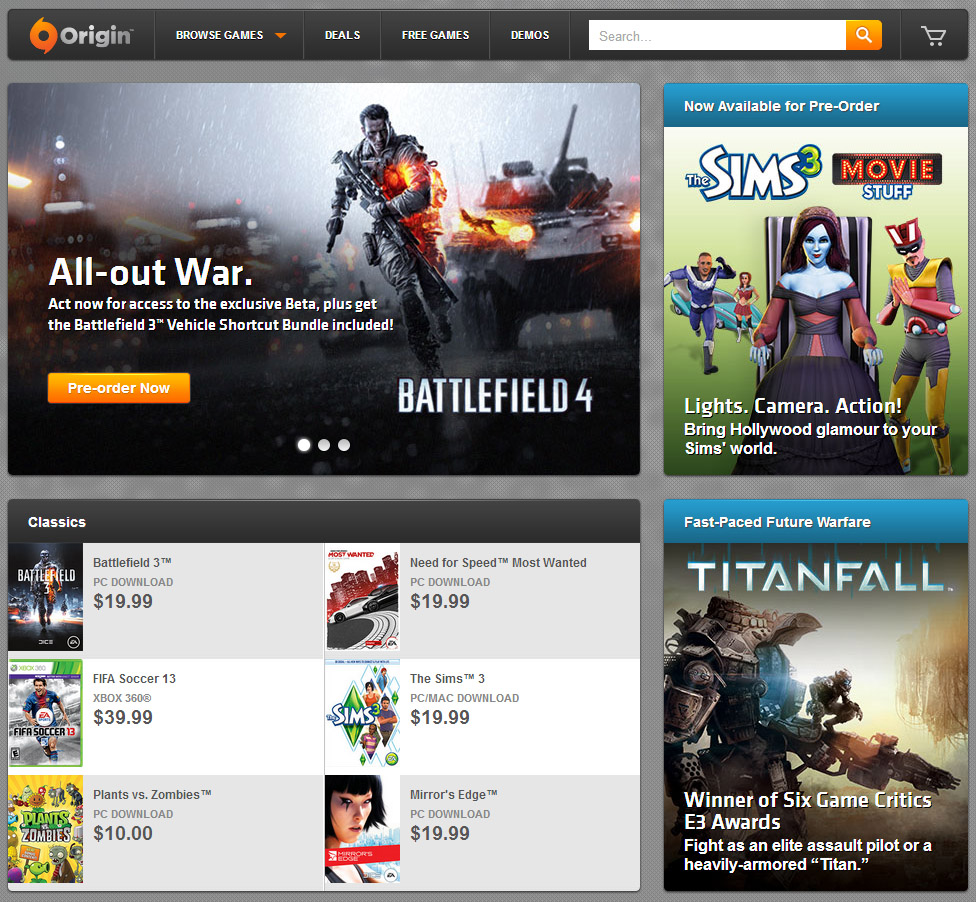This screenshot captures the homepage of Origin, a popular digital distribution platform for PC and console games. At the top, users are presented with navigation options to "Browse Games," "Deals," "Free Games," "Demos," a search bar with a magnifying glass icon, and a shopping cart feature.

Prominently featured is an advertisement for "Battlefield 4," showcasing an "All-Out War" theme. The ad urges users to pre-order to gain access to an exclusive beta and includes the "Battlefield 3 Vehicle Shortcut Bundle."

Adjacent to this is a promotional banner for "The Sims 3: Movie Stuff," highlighting the theme "Lights, Camera, Action" to bring Hollywood glamour to the Sims' world.

Another vibrant ad promotes "Titanfall," touting its fast-paced future warfare gameplay and its accolade of winning six Game Critics E3 awards. Players can engage as either elite assault pilots or heavily armored Titans.

Below these ads, a section titled "The Classics" displays popular game downloads along with their prices:

- "Battlefield 3" for PC at $19.99
- "Need for Speed Most Wanted" for PC at $19.99
- "FIFA Soccer 13" for Xbox 360 at $39.99
- "The Sims 3" for PC/Mac at $19.99
- "Plants vs. Zombies" for PC at $10
- "Mirror's Edge" for PC at $19.99

This comprehensive webpage offers a blend of promotional content and classic game listings, catering to a wide range of gaming interests on the Origin platform.